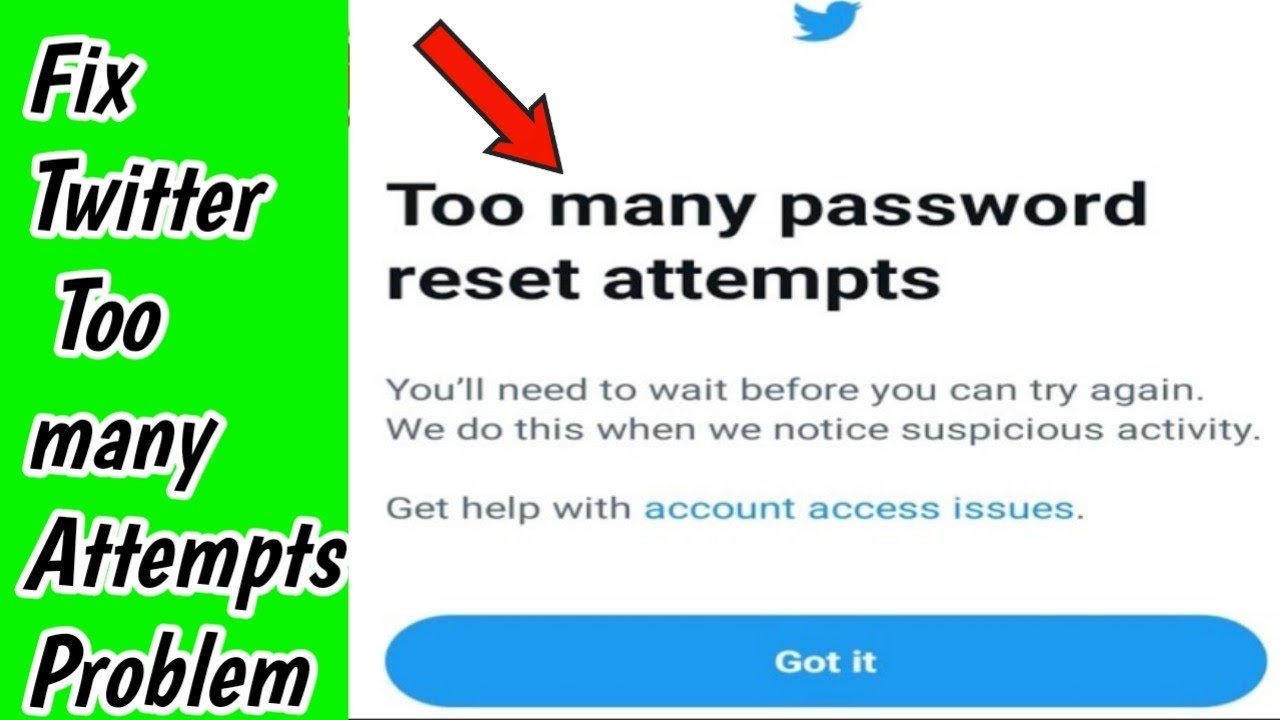**Image Description: "Too Many Password Reset Attempts" Error on Twitter**

The image is a screenshot likely taken from a digital interface, depicting a notification or error message associated with Twitter's account security measures. At the very top of the image, there is a prominent blue Twitter logo, instantly recognizable as the platform's official emblem.

Below the Twitter logo, there is a bold message in large, black letters stating, "Too many password reset attempts." A red arrow points downward from the top of the image, specifically targeting the "M" in the word "many," perhaps to draw attention to this section of the message.

Further down, additional text explains the situation: "You'll need to wait before you can try again. We do this when we know this is a suspicious activity." This message indicates that the account is temporarily locked due to multiple failed password reset attempts, which Twitter flags as potentially suspicious behavior.

Following this explanatory message, there is a hyperlink that reads, "Get help with account access issues," suggesting users click here for further assistance. Beneath this, a noticeable blue button with white text states, "Got it," likely allowing users to acknowledge and close the message.

To the left side of the screen, on a striking neon green background, there is sizable text in black letters outlined in white that says, "Fix Twitter Too Many Attempts Problem." This text spans the entire height of the box from top to bottom, making it highly visible and likely serving as a headline or informative prompt related to resolving the account lock issue.